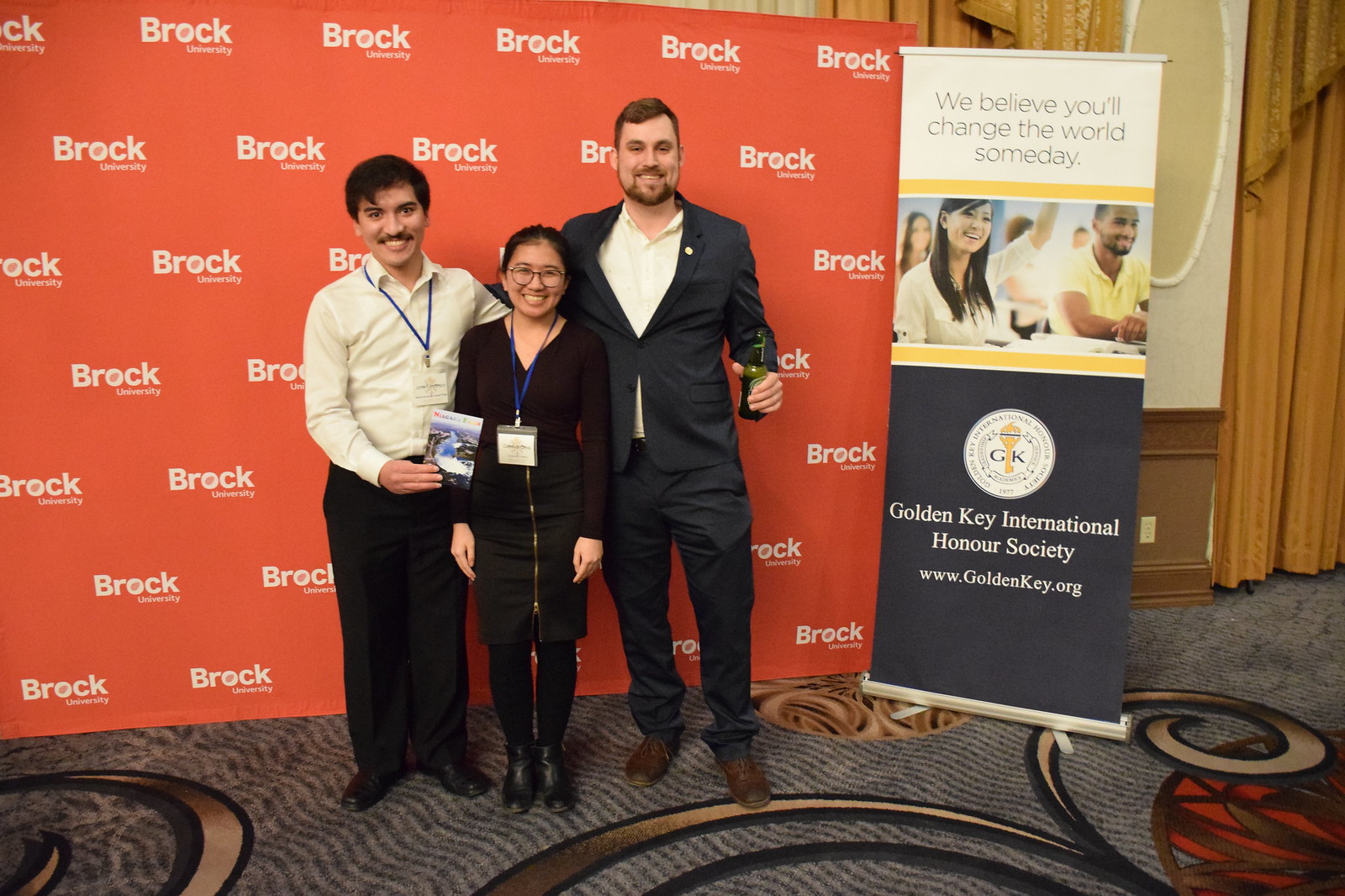In this photograph, three individuals stand prominently against a vibrant red backdrop that repetitively displays "Brock University" in white text. To their right, a tall, rectangular sign from the Golden Key International Honor Society features the inspirational message, "We believe you'll change the world someday," along with the society's emblem and website.

The individuals, dressed in business attire, appear to be honorees at a Golden Key International Honor Society event. The man on the left, sporting a mustache and black hair, is attired in black pants and shoes, paired with a white dress shirt. He wears a blue lanyard and holds a pamphlet, with his arm around the woman in the middle. She is the shortest of the trio, with black hair, glasses, and a black dress complemented by long black socks and black shoes. The man on the right, distinguished by brown hair and a goatee, is clad in a black suit, white undershirt, and brown shoes. All three have badges around their necks.

They stand on an ornate gray carpet with intricate gold spiral designs and wavy lines, creating an elegant setting for this commemorative moment. Their close positioning and interlocking hands on hips and shoulders highlight a sense of camaraderie and unity at this prestigious event.